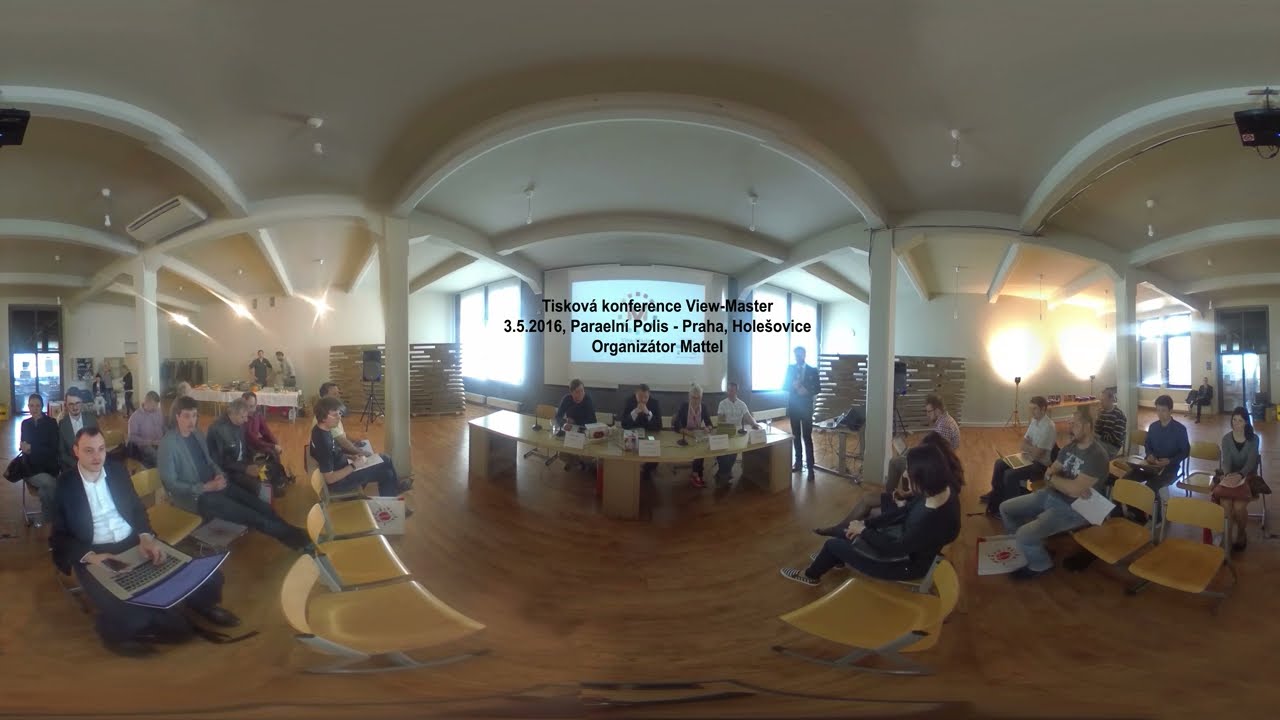The photograph is a panoramic, color image of an indoor conference, seemingly set in an Eastern European country based on the text displayed. The image combines three separate views using a fisheye lens, presenting the scene in landscape orientation with a noticeable curvature. Central to the composition is a curved desk with three men sitting and addressing an audience. Above them is an illuminated screen displaying the text: "TSCOBA Conference Viewmaster 3.5-2016 Paranili Polis Praha Holesovice. Organizer Mattel." The text is somewhat indecipherable but suggests a connection to a conference or presentation setting.

On the left side of the photograph, attendees are seated in yellow chairs, some with open laptops, indicating a possibly casual and interactive atmosphere. A man in a suit jacket and white shirt sits among them, absorbed in his computer. The right side of the image captures more audience members, some with folded arms, all attentively watching the speakers. The background reveals additional conference areas with people either waiting or listening to other speakers, highlighting the event's scale and layout. The colors range from yellow and beige to white, blue, gray, and black, adding to the realistic, photographic style of the scene. The setting is clearly daytime, suggesting an engaged, professional environment. The photograph richly detailed, captures both the dynamics of the conference and the interactions within.